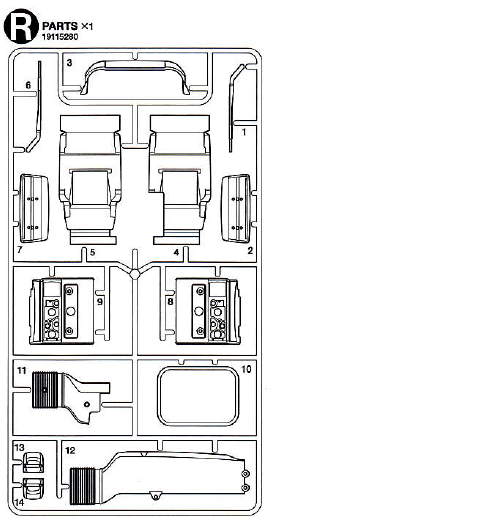This image is a detailed schematic or diagram featuring various numbered parts, potentially for a model car or air conditioning unit. The background of the image is white, with a line drawing that shapes an oblong vertical rectangle. In the upper left corner, there is a large uppercase white letter "R" inside a black circle. Adjacent to this circle in small black print, it says "Parts X1" followed by the numbers "19115280." The diagram contains 14 numbered parts, with part numbers 1 and 2 on the right side, numbers 3, 4, and 5 in the center, numbers 6 and 7 in the top left, numbers 8 and 9, 10, and 11 in the middle, and parts 12, 13, and 14 located at the bottom. Each part is clearly marked, although identifying the specific components or their functions is difficult from the image alone.